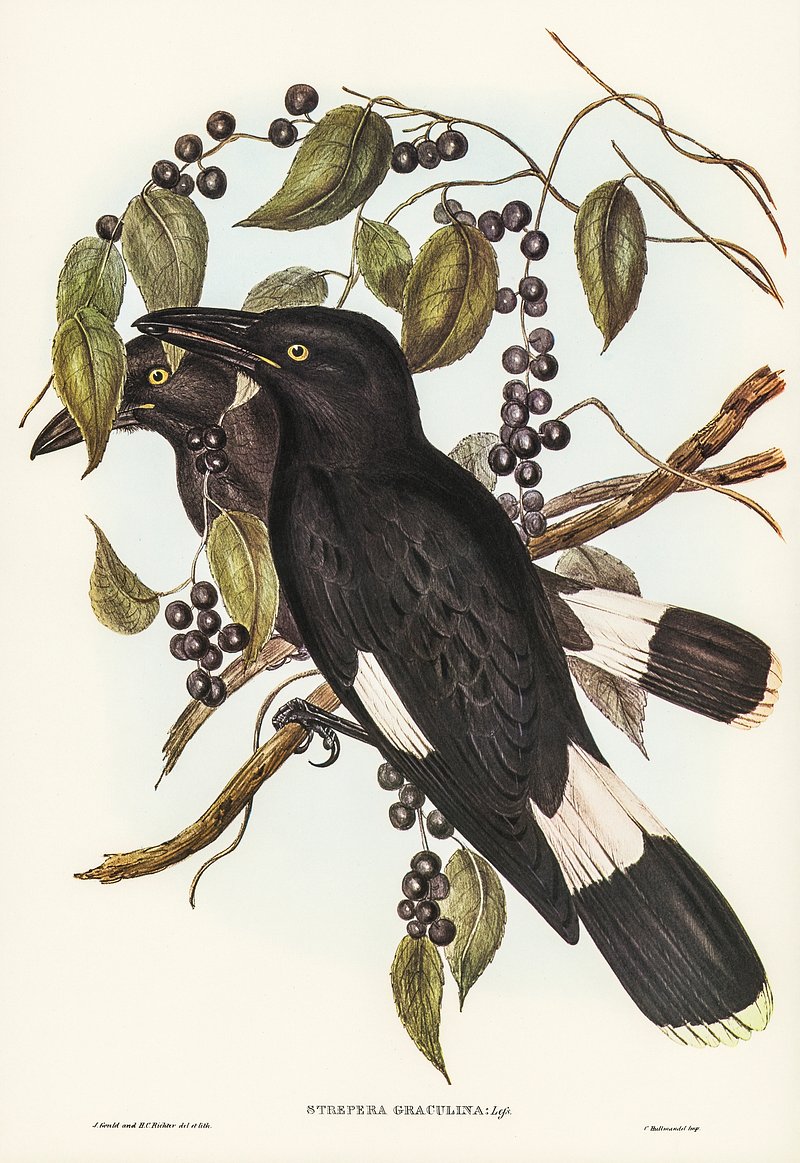This highly detailed color illustration portrays a pair of ravens perched on a tree branch adorned with olive green leaves and small black berries. The raven at the front is predominantly black with a glossy sheen, featuring white detailing near the tail and the tips of its wings. Its large black beak is slightly open, revealing a dark berry clutched within. Its striking yellow eyes with black pupils add a vivid contrast. Behind it, a second raven, slightly obscured and more brownish in hue, mirrors the same white tail and wing patterns. Both birds are perched on brown, diagonally positioned branches adorned with numerous stems bearing blackberries. Their gaze is directed to the left, adding a sense of unity in their posture. At the bottom of the image, partially legible text reads "streperagraculina LGS,” with additional cursive text at both the bottom left and right corners that is too small to decipher.